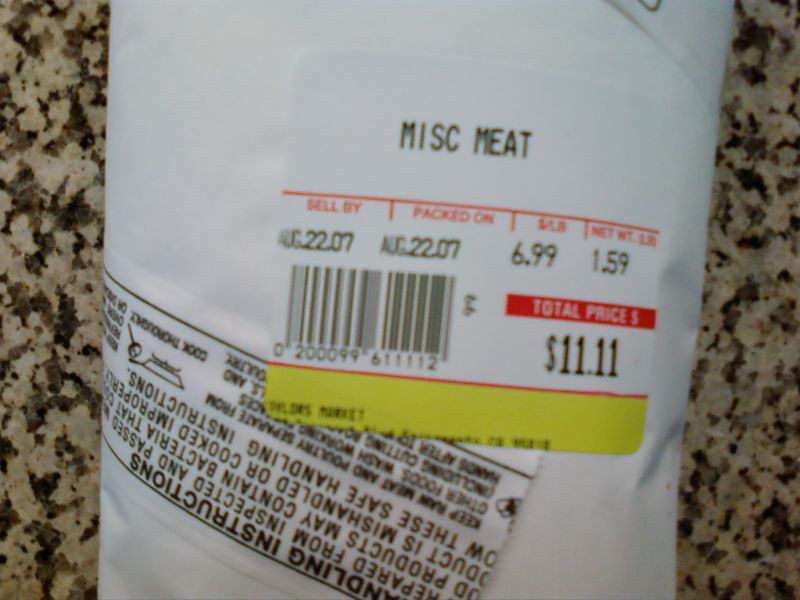In this close-up photograph, we see a packet of miscellaneous meat wrapped in white deli paper resting on an oatmeal and light brown granite-style countertop that’s speckled with greenish and beige spots. A sticker label on the package prominently reads "Miscellaneous Meat" in black letters against a white background. Beneath that, it details a sell-by and packed-on date of August 22, 2007. The label specifies the meat costs $6.99 per pound and weighs 1.59 pounds, resulting in a total price of $11.11 indicated in a red banner with white letters. To the left of this primary information, a barcode is visible along with some handling instructions on an upside-down label partially covered by the main label. Towards the bottom of the main sticker, a horizontal yellow band adds a touch of color.